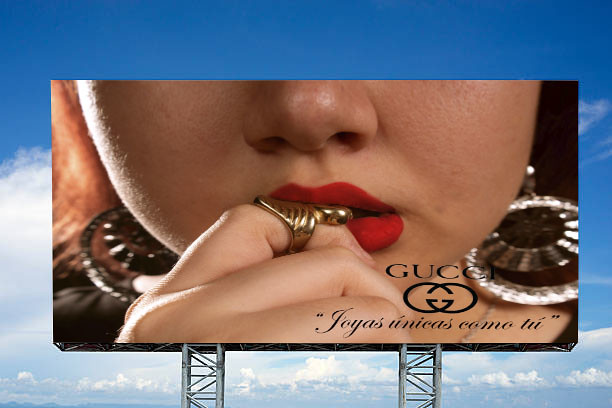The image depicts a rectangular billboard set against a blue sky with clouds. The main focus of the billboard is the lower half of a woman's face, featuring bright red lipstick and pale skin. Her hand, adorned with a large gold ring, is pressed against her lips, partially obscuring her mouth. She wears two large silver hoop earrings with an intricate inner layer of silver. In the bottom right corner of the advertisement, the Gucci logo is displayed prominently above their signature interlocking G's. Below the logo is the cursive Spanish phrase "Joyas únicas como tú." The image appears to be digitally rendered rather than a photograph, presenting an overall sophisticated and modern aesthetic.